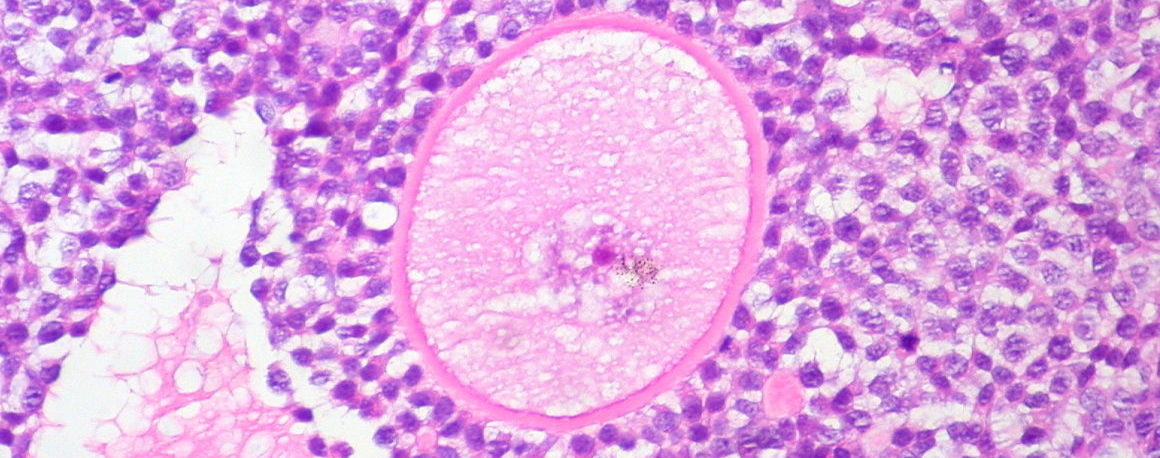The image appears to be a highly detailed, professional photograph, likely taken under a microscope for educational purposes, potentially from a medical or biology textbook. It showcases an intricate view at the cellular level, dominated by an array of colors, primarily various shades of purple, pink, and white. At the center of the image is a prominent spherical cell, clearly defined with a pink rim. This central cell contains dense areas of purple and white masses, resembling a nucleus surrounded by a diverse internal environment. Adjacent to the central cell, to the upper right, are notable concentrations of white matter, while a larger white and pink triangular form bends towards the bottom left. The background is filled with numerous purple specks and splotches, suggesting a rich, textured cellular or tissue environment.